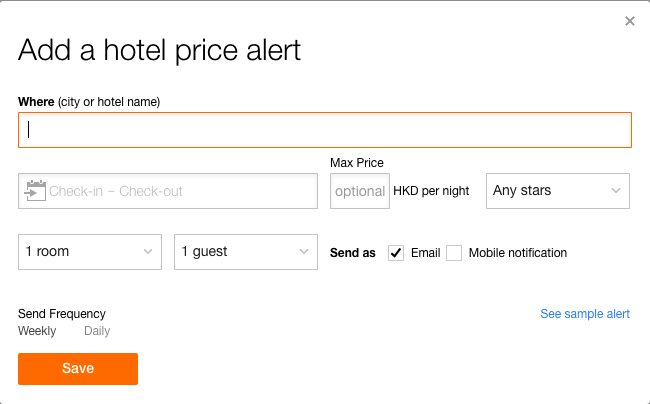This image illustrates a notification setup interface within an app, specifically designed for creating hotel price alerts. The interface appears as a pop-up window, identifiable by a thin black line at the top, while the other sides are not bordered. On the top-right corner, there's a gray 'X' icon to close the window. 

The heading "Add a Hotel Price Alert" is prominently displayed in black font. Directly beneath this heading, the section labeled "WHERE" in bold font requests the user to specify a city or hotel name, with an orange-highlighted input field provided for entry. 

Further down, another set of entry fields prompts the user to input check-in and check-out dates, along with an optional maximum price per night, denominated in HKD. 

The interface includes a filter option for hotel star ratings, allowing users to choose any number of stars. Another filter option enables selection of the number of rooms and guests, defaulting to one room and one guest.

For notifications, users can opt to receive alerts via email or mobile notification, with email being the preselected option. The notification frequency can be set to either weekly or daily.

Towards the bottom, an orange "Save" button is prominently displayed to finalize settings, while a "See Sample Alert" option in blue is available in the bottom right-hand corner for users to preview a sample notification.